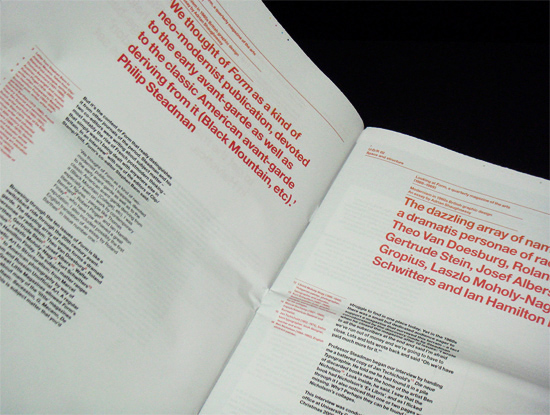This image features an open booklet or program, set against a black background. The booklet consists of two white pages with mixed red and black text. The left page contains a prominent red section reading, "We thought of Form as a kind of neo-modernist publication devoted to the early avant-garde as well as the classic American avant-garde deriving from it, Black Mountain excess, Philip Steadman." Below this is a small red paragraph followed by three smaller black paragraphs. The right page features another red header that states, "The dazzling array of a dramatist personae of Theo van Doesburg, Gertrude Stein, Josef Gropius, Laszlo Moholy-Nagy, Schwitters, and Ian Hamilton," accompanied by a small red paragraph and three small black paragraphs. The legibility of the finer black text is limited.